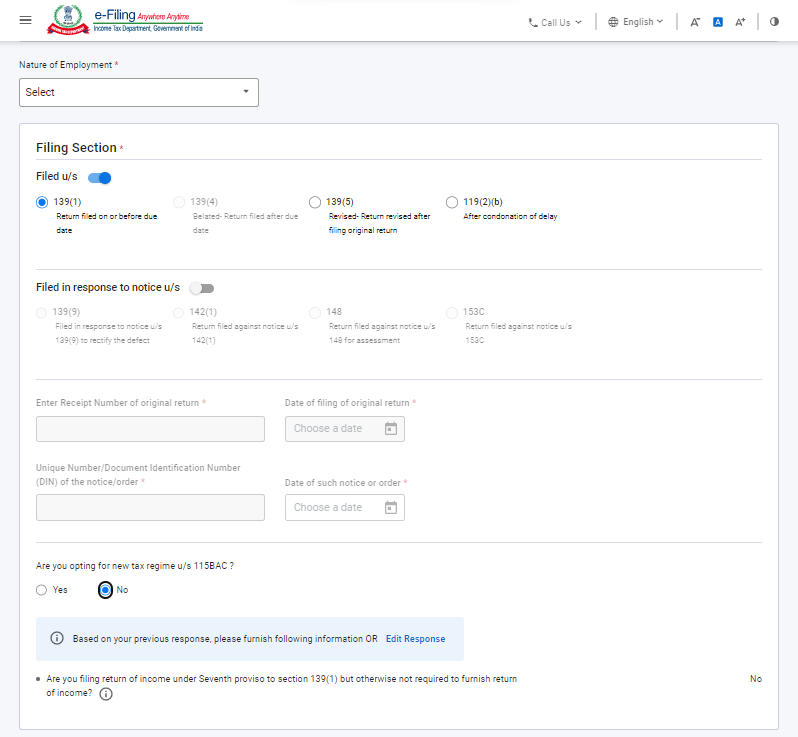Caption: Government of India's E-Filing Webpage for Taxes

This image showcases the Government of India's e-filing webpage, designed for seamless tax filings anywhere and anytime. In the top-left corner, there is a context menu next to the logo, featuring a useful pull-down menu. Users can access options like different font selections, along with night and dark modes. The main section is dedicated to various employment filing categories including form 1391 for returns filed before the due date, and revised returns filed under form 1192 after the original submission. Additional filing options include responses to notice U/S with other sections like 139(1), 142(1), 148, and 153(C). 

There is an input area for entering recipient numbers and document identification numbers at the bottom. A specific query asks users if they wish to opt for a tax regime under section 115BAC. Based on the input, users are prompted to furnish relevant documents or responses. Another section inquires whether the return filing is due to income earned after the 7th revision of section 1391, or if it is not required. The overall layout depicts a complex yet comprehensive tax filing form tailored for Indian citizens.